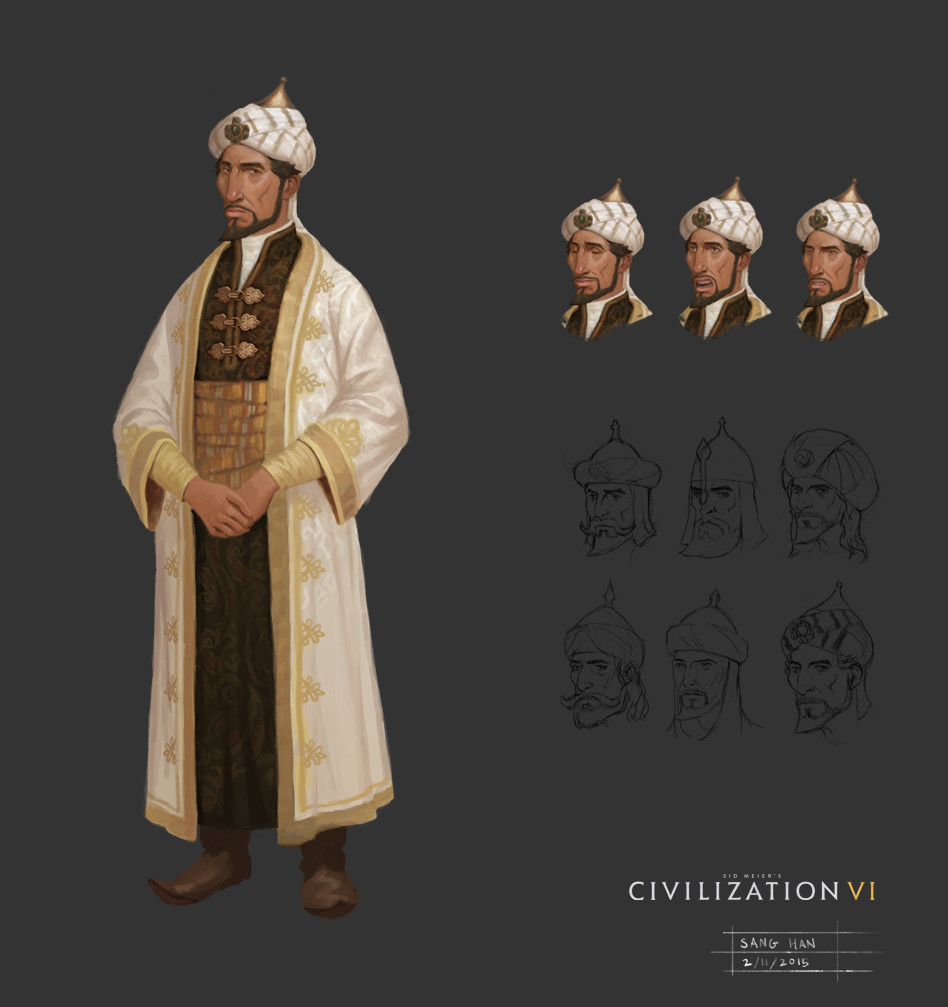The image is a detailed drawing of a man depicted in the video game Civilization VI, with the title written in white and the Roman numeral VI in a gold color at the bottom right-hand corner. The man, who appears to be of Middle Eastern or Indian descent, is dressed in traditional attire. He wears a white turban adorned with a metal comb-shaped decoration at the pointed top. He has brown hair, a brown mustache, and a brown goatee. His primary outfit includes a beige robe with pale golden trim, and underneath, he dons a long brownish-black dress with six buttons on the chest and a thick, lighter brown belt. His feet are clad in brown, pointed boots. He has both hands folded in front of his tummy and is looking towards the right of the image. 

The background is a dark gray, and to the left, from top to bottom, you see a full-body sketch of the man. To the right, there are three colored portraits of his head, showing different facial expressions. Below these, there are three rows of sketch drawings portraying various headshots of men in similar hats and beards. At the bottom of the image, it says "Civilization VI" with a date, 2-11-2015, and some smaller, less readable text. The scene evokes a historical setting, reflecting a detailed blend of artistic character design for the game.